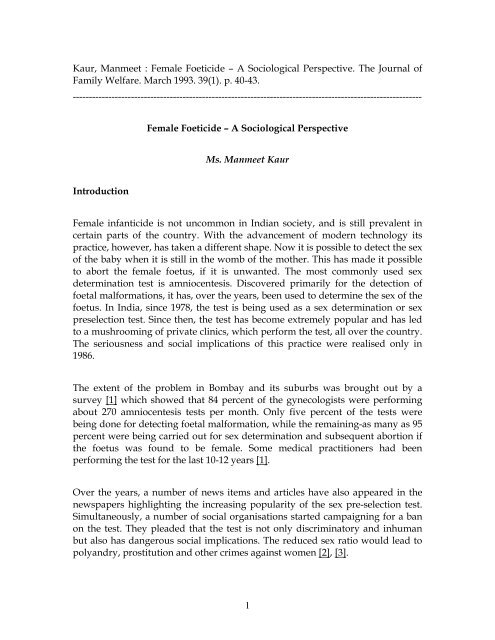The image displays a scholarly article excerpt formatted as black text on a white background, consisting of three paragraphs under the main heading "Female Feticide: A Sociological Perspective" by Miss Manmeet Kaur. At the top of the document, there is a citation indicating its source: "The Journal of Family Welfare, March 1993, pages 40-43." The introduction discusses the continuing issue of female infanticide in Indian society, which has evolved with modern technology into the practice of female feticide. It explains that prenatal sex determination tests, originally developed for identifying fetal malformations, have been widely used in India since 1978 to detect the sex of unborn babies. This practice has led to an increase in abortions of female fetuses, facilitated by the proliferation of private clinics offering these services. The societal implications and seriousness of this trend began to be recognized in 1986. The document appears to be the first page of this journal entry, detailing the sociological impact of female feticide in India.